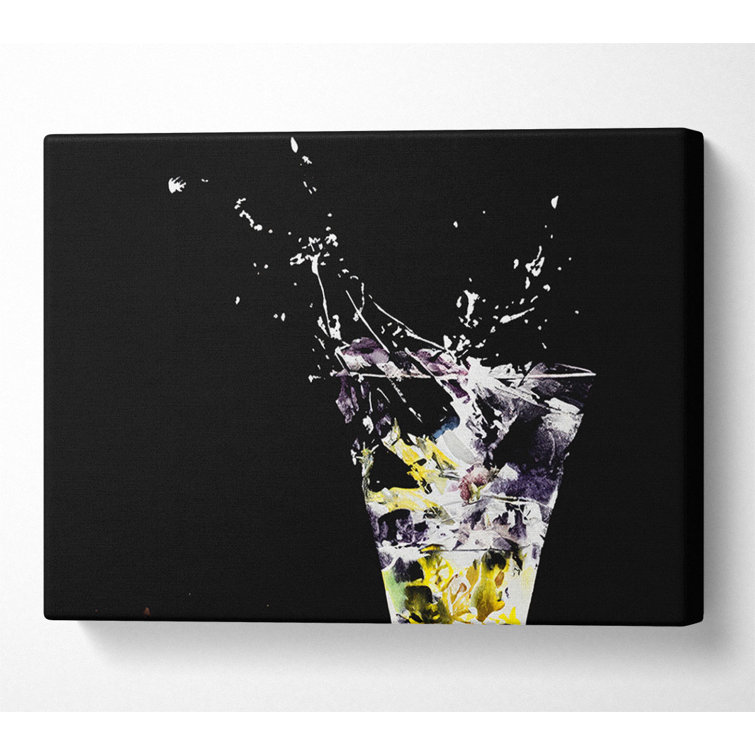The artwork, a photograph of a painting displayed on a white wall, rests on a black, unframed canvas that wraps around the edges. The piece features a clear, fluted glass, narrower at the bottom and flaring towards the top, although the stem or foot is not visible as it is cropped out of the frame. The glass appears filled with ice and a translucent liquid, possibly an alcoholic drink like a martini. There are greenish objects that resemble olives among the ice. The focal point of the painting is the dynamic splash of liquid and ice erupting out of the glass, creating a vivid sense of movement. This splash is rendered with white and yellow hues, and hints of purple, suggesting the liquid's shimmering motion against the stark black background. The painting's overall style leans towards impressionist or abstract, with noticeable brushstrokes contributing to its textured and lively composition.